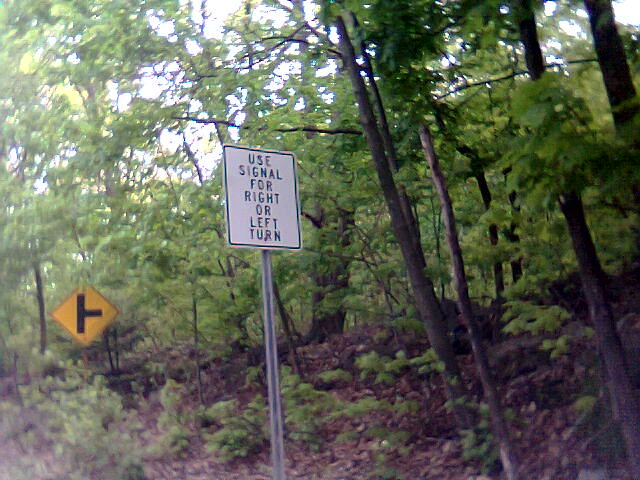The photograph captures a dense forest scene viewed from a roadside, featuring two prominent traffic signs amidst the greenery. Dominating the center of the image, a white sign mounted on a gray pole instructs, "USE SIGNAL FOR RIGHT OR LEFT TURN" in bold, black capital letters. This sign stands out clearly against the muted tones of the forest backdrop and fallen leaves that cover the brown, soil-rich ground. To the far left of the picture, a yellow diamond-shaped sign near the bottom third of the frame indicates an upcoming right turn with a black T figure and the stem pointing right. The scene is bright yet somewhat muted, with the light filtering through the green leaves of young trees, possibly oaks, allowing glimpses of the sky, particularly in the top left corner. Shadows on the forest floor suggest a sunny day, adding a subtle play of light and dark to the overall composition.